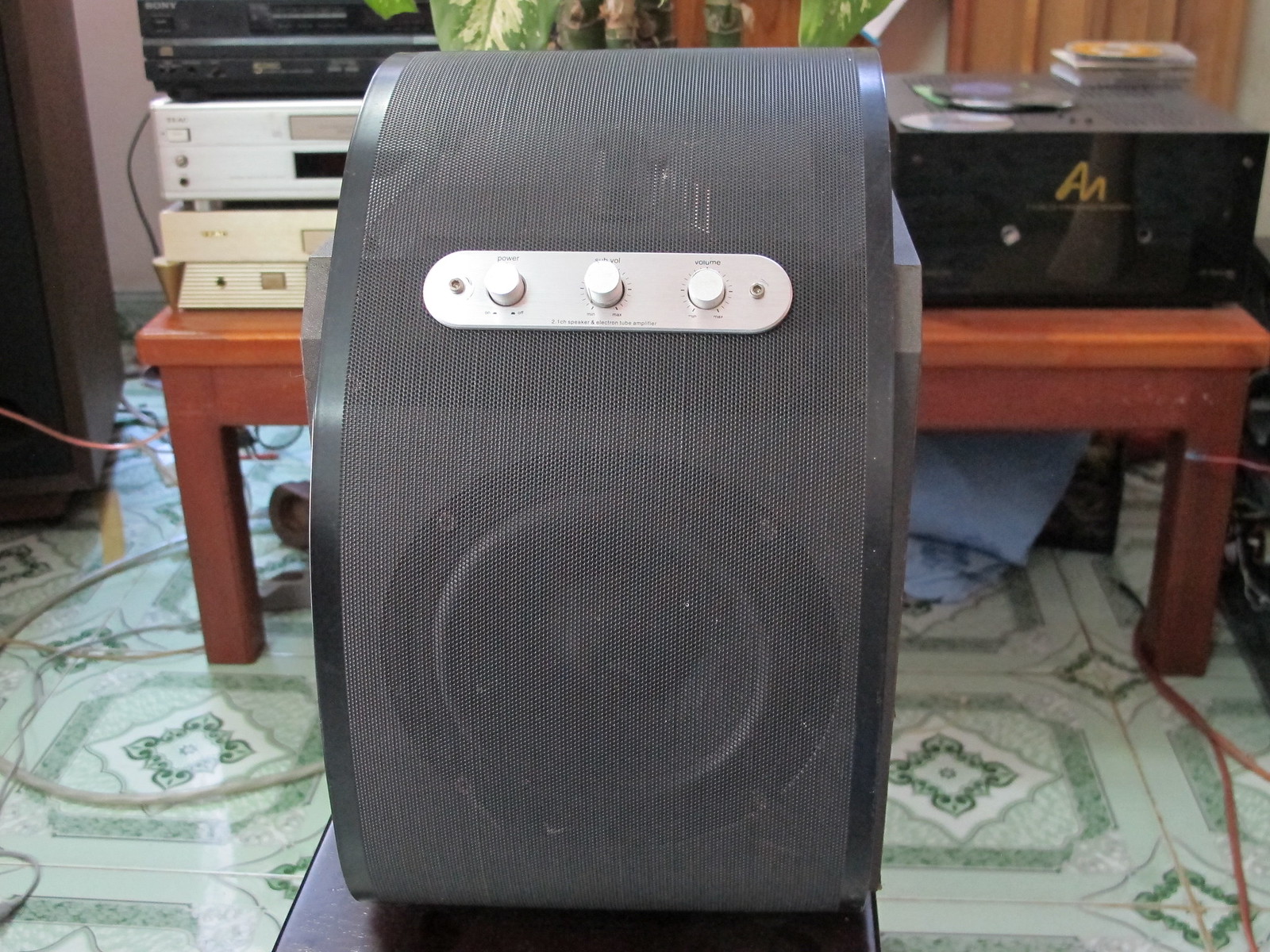The indoor photograph depicts a black speaker system positioned centrally atop a black elevated surface amidst a living room setting. The speaker features a black mesh cover, partially transparent, revealing a round subwoofer and several shiny black strips. Centrally, a horizontally laid oval panel, silver or light gray in color, houses three control knobs, each marked with notches. Text labels near the knobs include "power" and "volume." The base of the speaker structure includes a dark brown stand. The floor beneath is intricately designed with porcelain tiles, showcasing floral patterns within squares. In the background stands a low, red wooden coffee table laden with numerous electronic devices, including a VCR, CD player, mixer, and a closed video player.